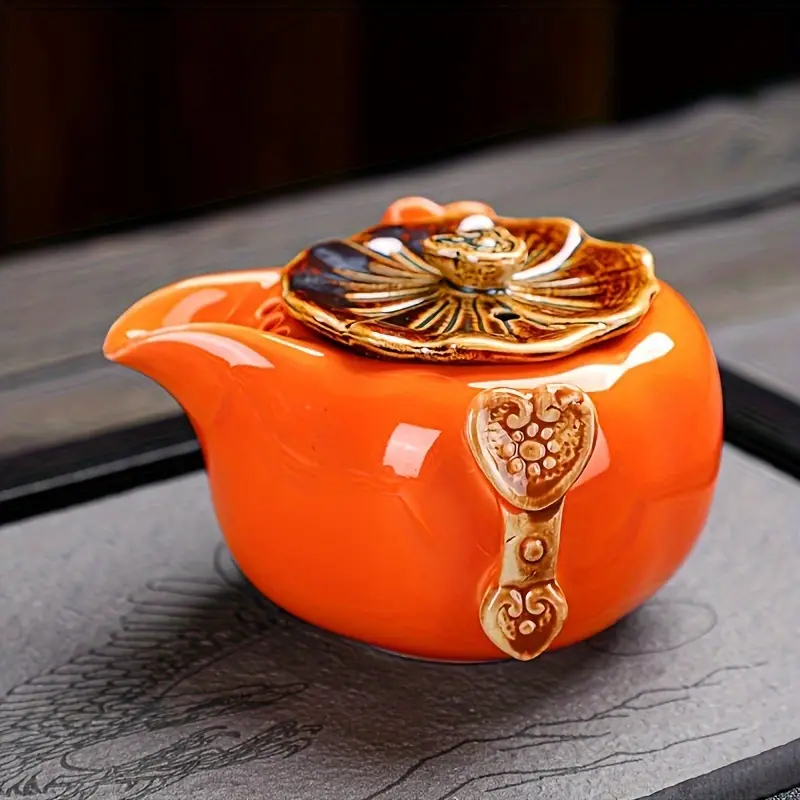The image depicts a vibrant, solid bright orange teapot with a short, round, kettle-like design, devoid of a handle. The teapot has a spout for pouring and features dark brown decorations, including an engraved flower and heart motif. Its circular lid is a mix of brown and dark brown, adorned with a small goldish-brown knob that matches a similar decoration on the teapot's body. The teapot, which has a shiny finish that reflects light, is positioned with its spout facing left and sits atop a gray stone surface that bears intricate carvings. The background is a blend of a slightly blurry gray, resembling wood, and a solid black area in the upper left part of the image, adding depth to the scene.